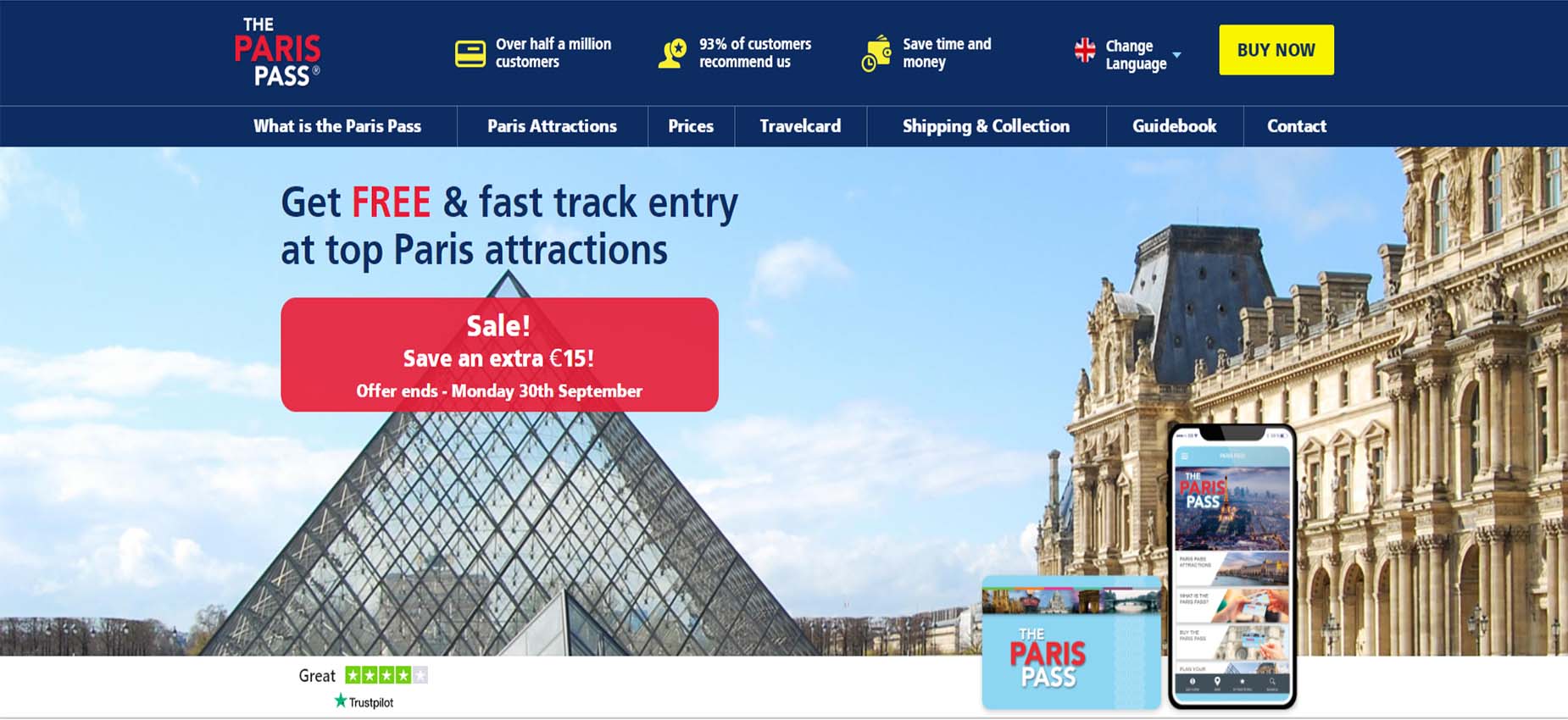The screenshot depicts a promotional advertisement for "The Paris Pass." The background is a gradient dark blue at the top, transitioning to lighter shades downward. On the upper left-hand side, "The Paris Pass" is prominently displayed in white text, with the word "Paris" highlighted in red. Centrally positioned in the right half of the image, we see a series of white text stating, "Over half a million coasters. 93% of customers recommend us. Save time and money." 

In the top right corner, there is an option to change the language, indicated by a British Union Jack, symbolizing the English option. Beneath it is a blue "Buy Now" button outlined in a yellow rectangle.

The main visual features an outdoor scene with the iconic glass pyramid of the Louvre Museum prominently displayed in the foreground. Blue text at the center states, "Get free and fast track entry at top Paris attractions," with "FREE" written in bold red letters. To the right, several older, classical Parisian buildings with creamy white facades and gray roofs are visible, reinforcing the Parisian atmosphere.

Embedded in the visual are images of a smartphone and a light blue card, both displaying what appears to be "The Paris Pass," emphasizing its digital and physical availability.

The overall design is clean and straightforward, effectively promoting the benefits of The Paris Pass to potential tourists.